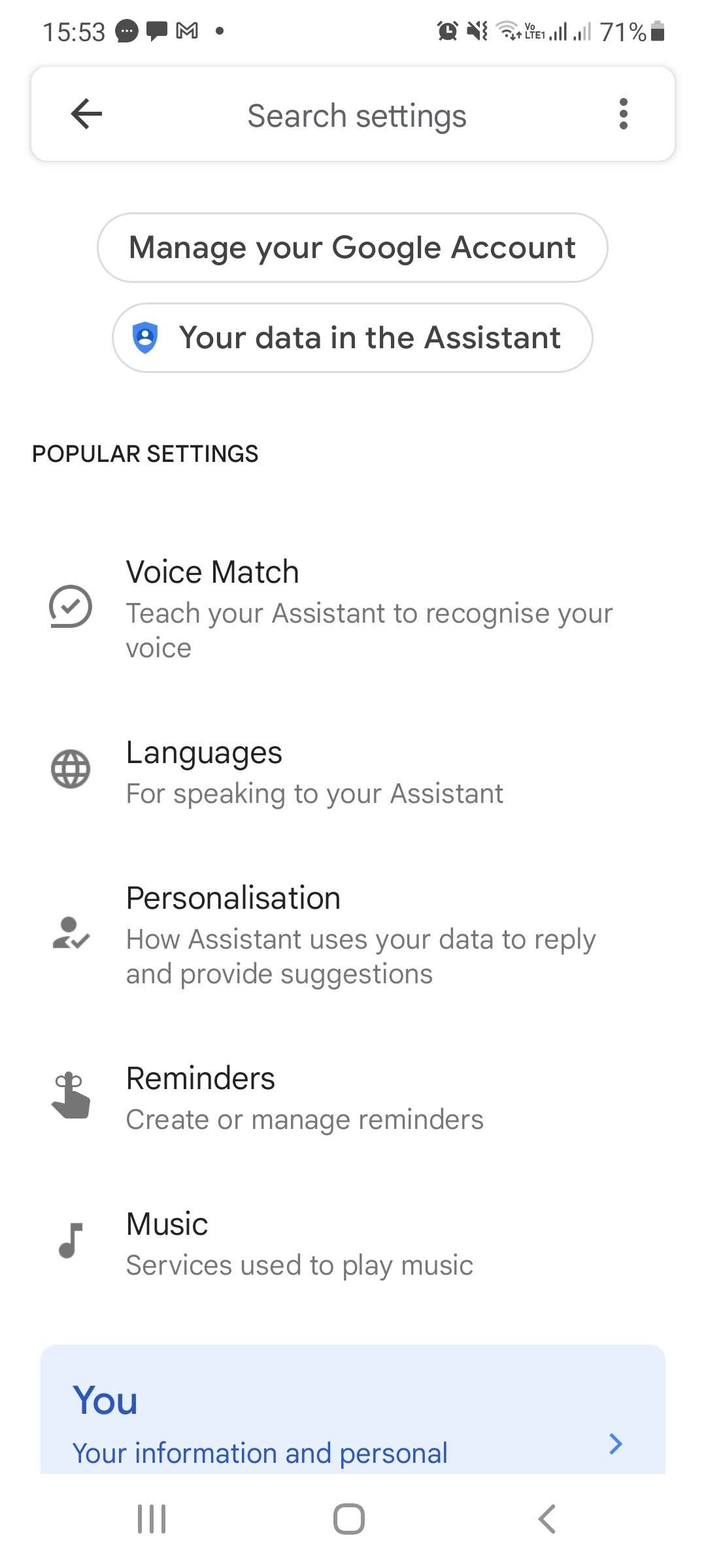The image displays a smartphone screen showing the Google Assistant settings menu. At the top of the screen, the status bar indicates it is 15:53, with chat notifications, Gmail alerts, and a silent alarm mode active. The device is connected to Wi-Fi with full bars and LTE signal strength showing two bars, and the battery is at 71%.

Below the status bar, the top navigation includes a back arrow, a search icon, and three vertical dots for more options. The main section features several settings categories, starting with "Google Account" next to a blue shield icon. Following this, there are "Popular Settings," including "Voice Match," which prompts users to teach the Assistant to recognize their voice, marked by a globe icon for language settings.

The "Personalization" section is marked with a silhouette and a check symbol, indicating how the Assistant uses data to provide replies and suggestions. "Reminders" are represented by a finger with a circular icon, guiding users to create or manage reminders. The "Music" section, labeled with a musical note, relates to services used to play music.

At the bottom of the screen, navigation options include a right-facing arrow, three horizontal lines, a square, and a back arrow, facilitating easy movement through the device's interface.